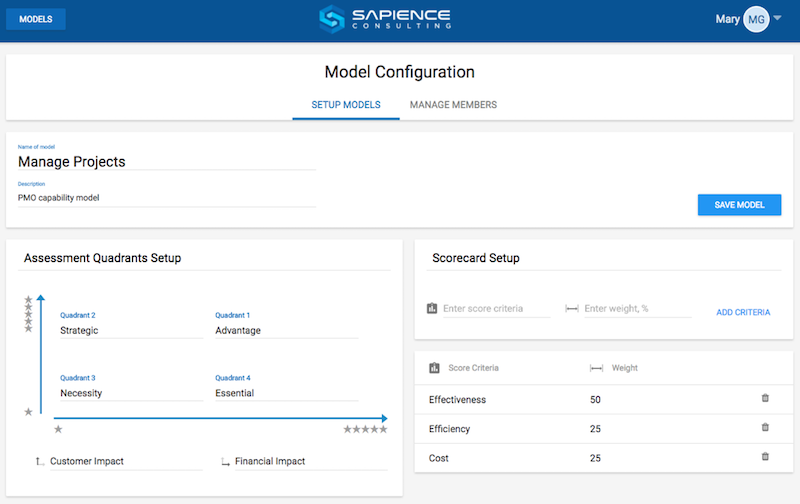The image features a blue background with detailed content related to model configuration and consulting. At the top, the title "Models" is displayed on the left-hand side, while the center prominently features the text "SAPIENCE Consulting." On the right-hand side of the image, a figure named "Mary" is visible.

In the center, there's a white circle with the initials "M"G" in blue text. Below this, the words "Model Configuration" appear in black, with "Setup Models" in underlined blue text underneath. Following this, there are additional options listed in blue text: "Manage Memberships," "Manage Projects," and "PMO Capability Model."

On the right-hand side, a blue rectangle contains the text "Save Model" in white. Below this, the section titled "Assess Quadrant Setups" includes a blue upward-pointing arrow and a blue rightward-pointing arrow, along with five gray stars situated near the arrows and two additional gray stars positioned in the bottom left.

The image further includes several descriptive terms and metrics: 
- "Strategic Advantage," "Density," and "Necessity Essential" are written in black text.
- "Customer Impact" and "Financial Impact" are mentioned as key factors.
- Specific aspects such as "Store Card Setup," "Effectiveness," "Efficiency," and "Cost" are listed, each accompanied by numerical values: 20, 50, 25, and 25 respectively.